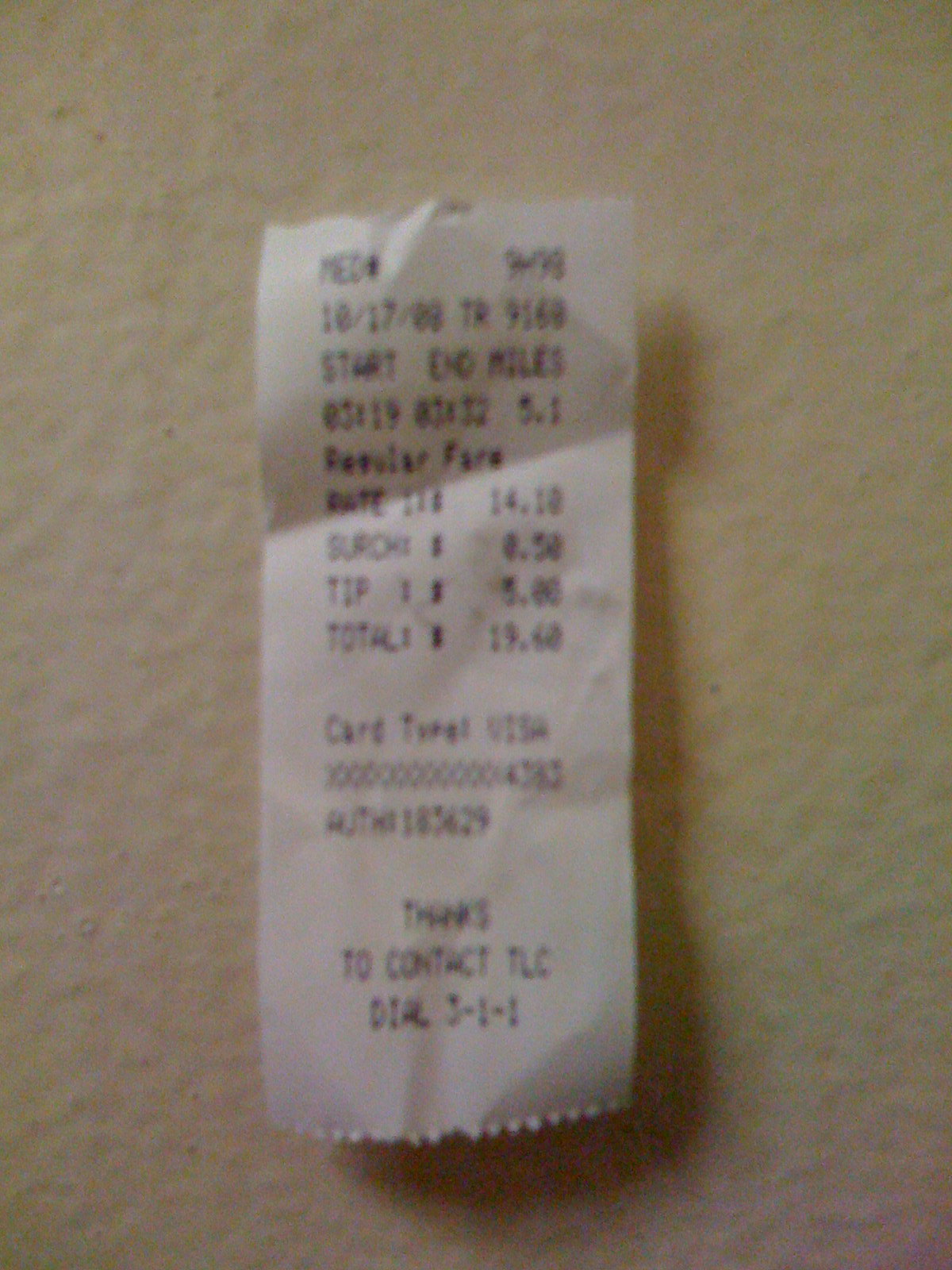This photograph captures a low-quality, grainy image of a blurry paper receipt placed against an off-white painted surface, possibly a wall or floor. The receipt itself is printed on white paper with black text that is largely unreadable due to the quality of the image. At the bottom of the receipt, some text can be discerned, reading "thanks to contact TLC," along with some illegible digits. The itemized details are mostly indistinguishable, though the term "regular fare" is somewhat visible. Additionally, there is a date and time stamp present on the receipt, alongside references to "start and end miles," suggesting that this might be a receipt for a transportation journey.